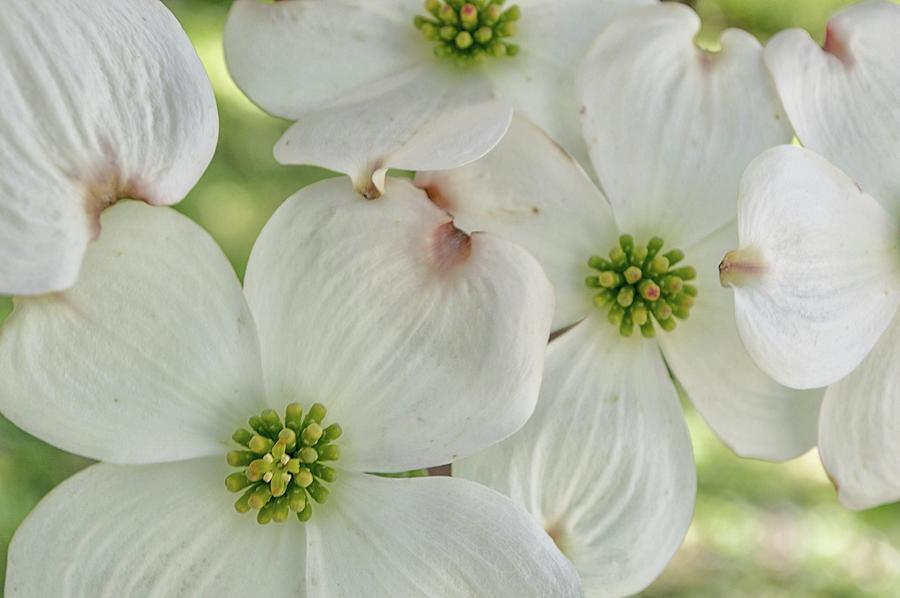This is a close-up, rectangular color photograph predominantly capturing a cluster of white flowers, set against a muted, blurry green background, suggesting an outdoor setting, possibly a grass field. The image prominently features flowers with four heart-shaped petals that are white with pinkish-brown tips, indented as if a small notch has been taken out, adding a unique texture to each petal. 

In the composition, there is a large flower petal starting from the top left corner, while two nearly complete flowers occupy the center. Another flower descends from the top, and one more is partially visible on the right side. Each flower showcases a central bundle of short green spindly structures, giving a detailed view of their blooming state. The arrangement draws the viewer's eye to the intricate and delicate features of the petals and centers, providing a vivid, intimate look at these blossoms.